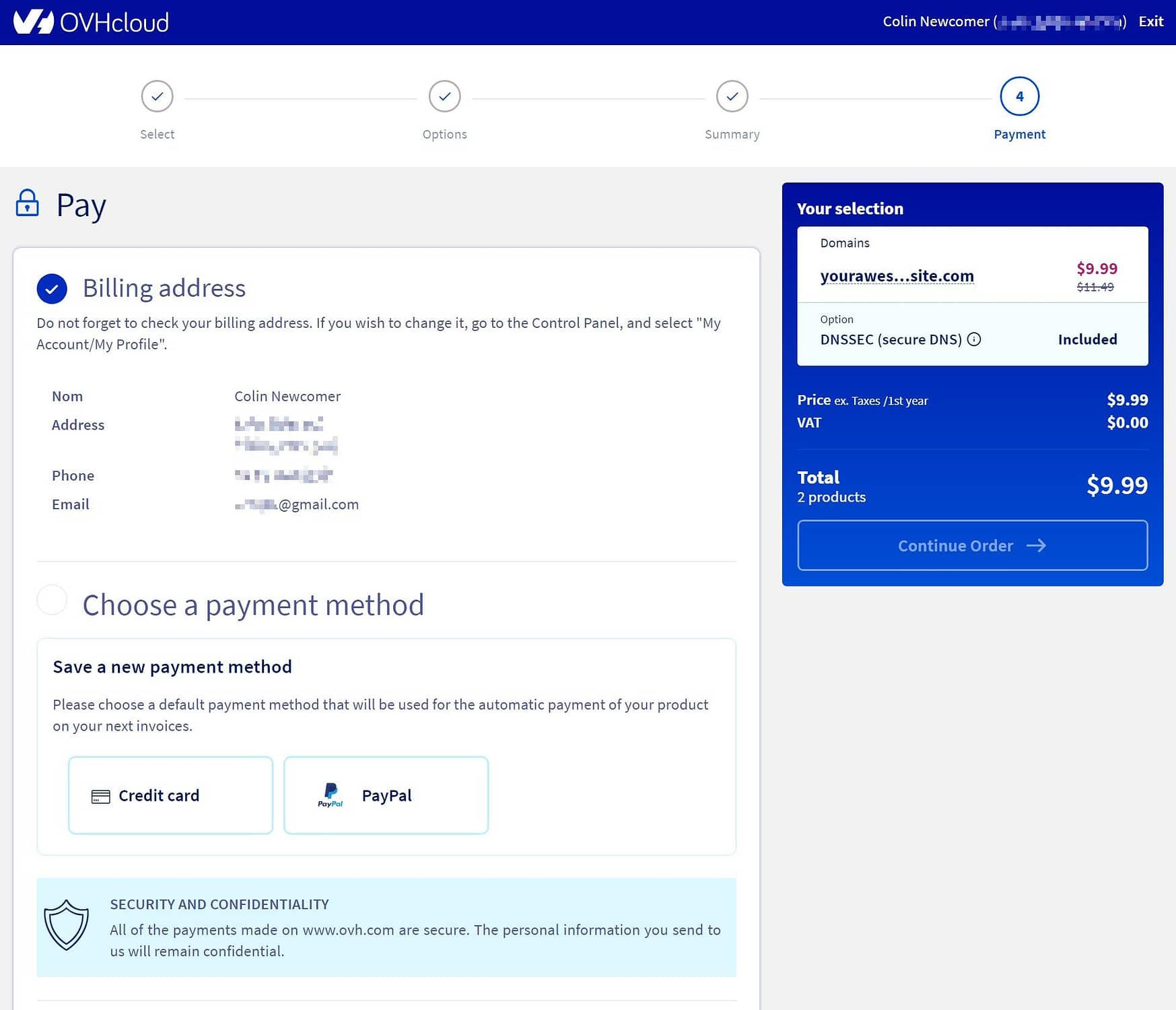The image is a screenshot of a web page, presumably from a computer, displaying a payment section for a service or product from the company OVH Cloud. At the top, a blue horizontal banner stretches across the full width of the page. On the left side of the banner, in white letters, "OVH cloud" is written, with "cloud" notably in lowercase. An emblem, likely the company's logo, appears adjacent to the text.

On the right end of the same blue banner, there is a column labeled "newcomer," though this term is marked out and rendered illegible. Adjacent to it is the word "exit."

Below the banner, a navigation menu presents several options: "Options," "Summary," and "Payment." The "Payment" tab is highlighted, indicated by a blue circle containing the number 4 and the word "Payment" underneath.

The main section of the page is dedicated to the payment process. A light gray box features the word "Pay" in white text. Below this box is a section for the billing address, marked by another blue circle with a white checkmark. Accompanying text advises the user not to forget to verify their billing address and provides instructions for changing it via the control panel under "My Account" and "My Profile."

The billing address section displays the name "Column Newcomer" and placeholders for the address, phone number, and email, all of which are blurred except for the domain "gmail.com."

Further down, users are presented with options to save a new payment method, choosing between a credit card and PayPal. A banner concerning security and confidentiality is also visible. The selected service's price appears at the bottom, listed as $9.99, summarizing the total charge.